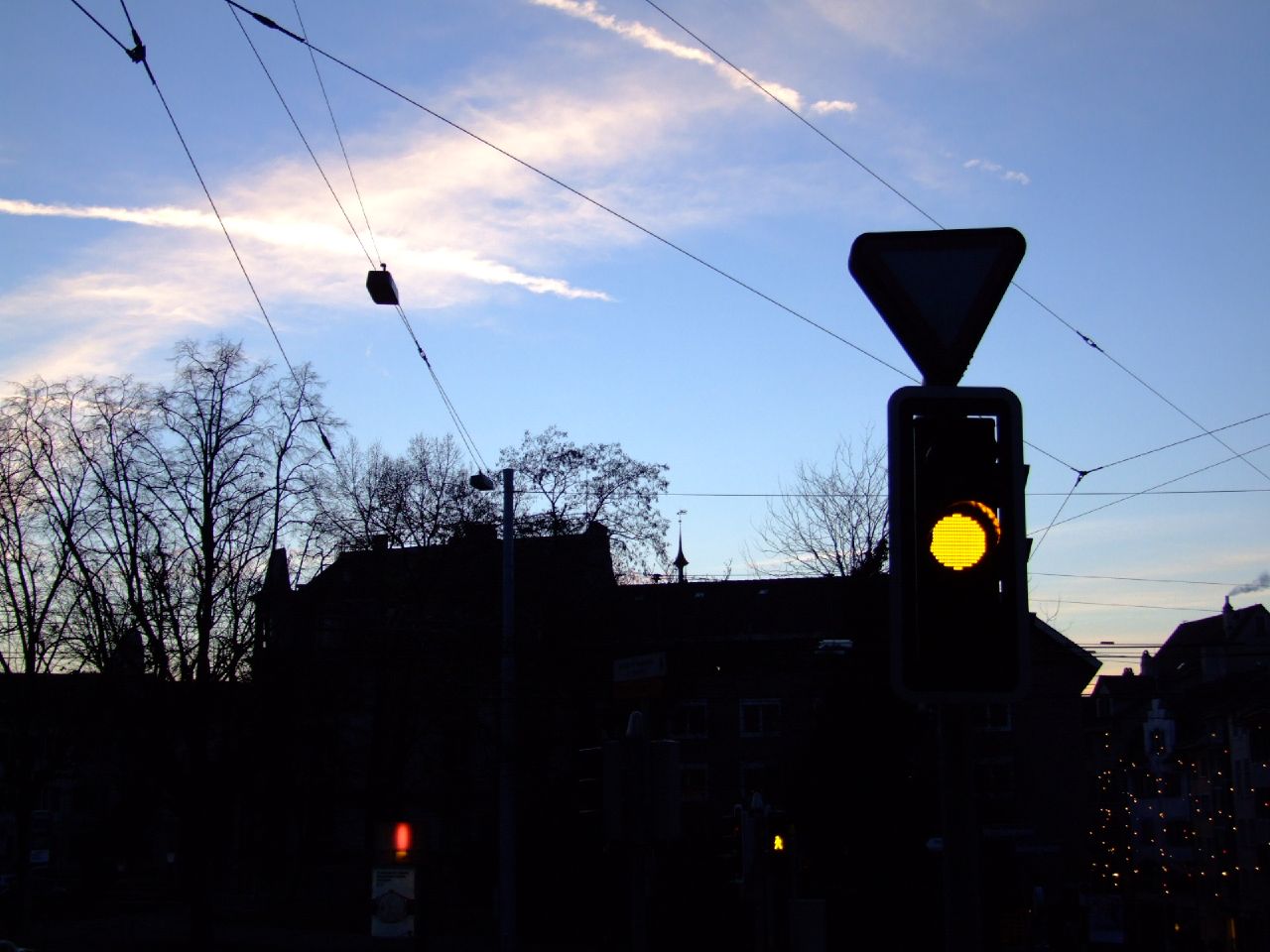A captivating photograph captures a city skyline under a bright blue sky adorned with delicate, wispy clouds drifting to the left. Streaks of white cloud the sky, partially obscuring a subtle yellowish glow. In stark contrast, the lower half of the image is dominated by silhouetted elements. Trees in the background are depicted as dark shapes, with branches starkly devoid of leaves. The black outlines of rooftops from nearby buildings contribute to the urban landscape. In the foreground, to the right, a traffic light stands out with a triangular sign perched above it, emitting a warm yellow glow that adds a touch of urban life to the serene skyscape.